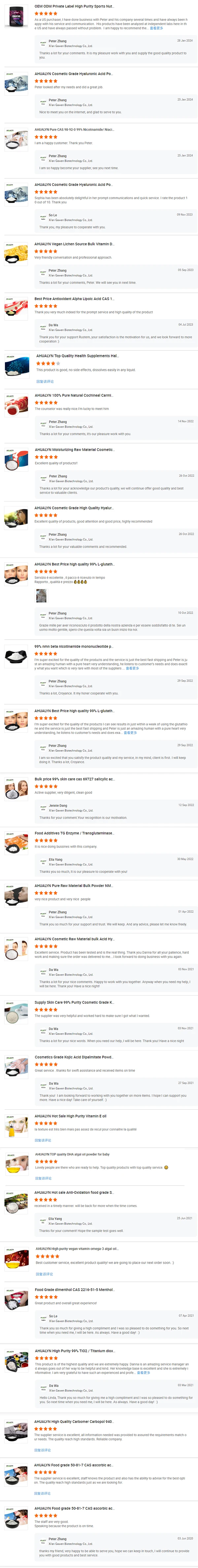The image depicts a computer screen showcasing a product catalog. On the left side of the screen, there are elongated thumbnails of various products, with a number of images featuring faces or pairs of faces, possibly demonstrating the use of facial care items such as powders or solutions. The pictures are arranged in a vertical column. On the right side of the screen, each product listing includes a star rating, with all items receiving five stars. Beneath each star rating, brief product descriptions are visible, typically consisting of a few sentences. This layout helps consumers to quickly assess and compare different products, based on their ratings and descriptions.